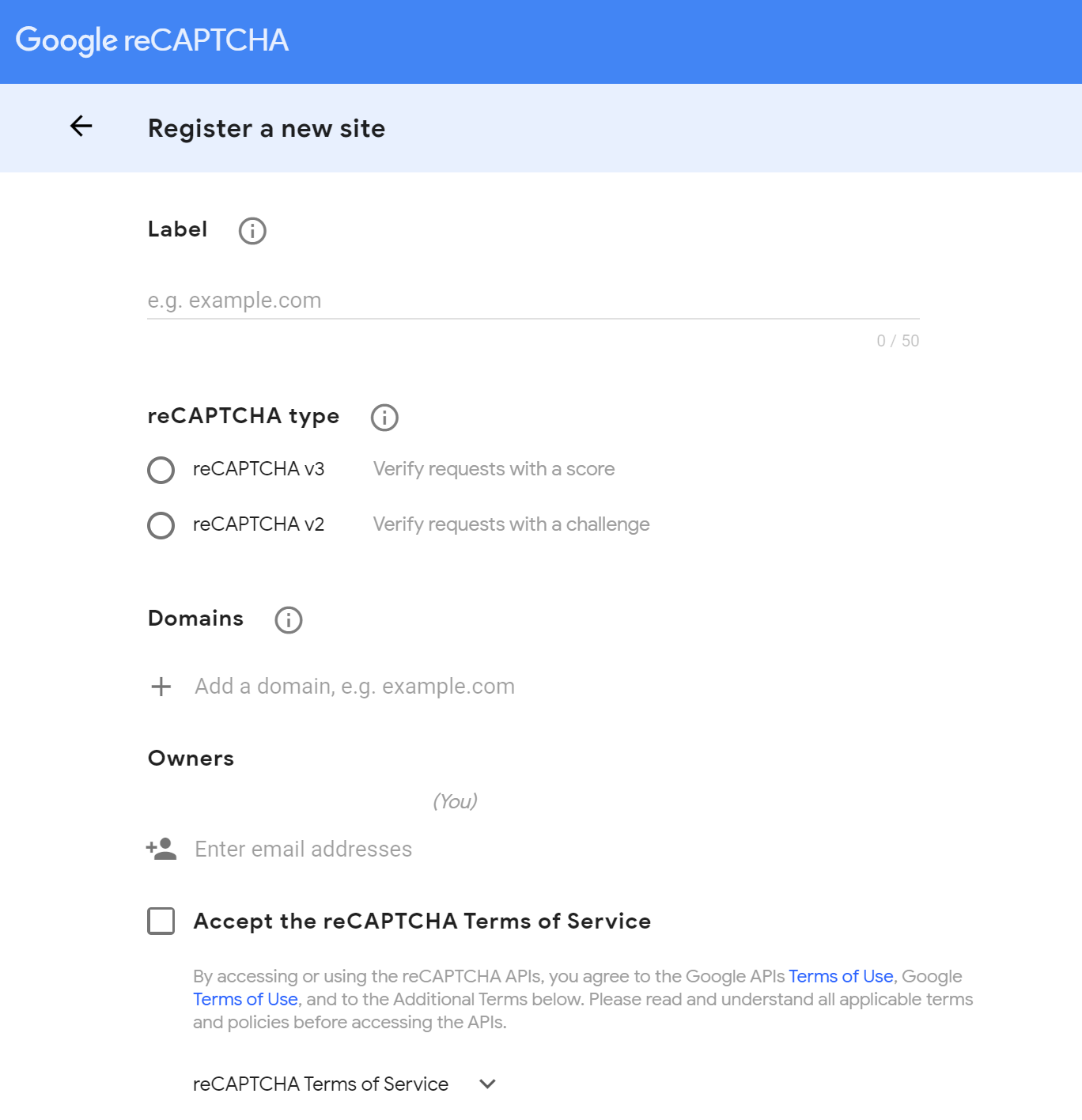---
**Web Page Screenshot: Google reCAPTCHA Registration**

At the top of the captured web page, there is a prominent bright blue banner featuring the Google "reCAPTCHA" logo. The word "Google" is displayed in white, while "reCAPTCHA" follows with "re" in lowercase and "CAPTCHA" in uppercase letters.

Just below this, there's a pale gray banner that reads "Register a new site" in bold font, followed by a left-pointing arrow.

The main body of the page is white and organized into several sections:

1. **Label**: 
   - Accompanied by an information (i) icon, this section includes a text box with the placeholder "example.com" where users can enter a label for their site.

2. **reCAPTCHA Type**: 
   - This section, also featuring an info button, offers two radio button options:
      - **reCAPTCHA v3**: Verifies requests based on a score.
      - **reCAPTCHA v2**: Verifies requests using a challenge.

3. **Domains**: 
   - Comes with an information (i) icon and an option to add domains with a plus (+) sign. The example domain shown is "example.com."

4. **Owners**: 
   - Users can input email addresses of owners in this section.

5. **Accept Terms of Service**:
   - A checkbox here allows users to accept the reCAPTCHA Terms of Service. The terms are accessible through a dropdown box for more detailed reading.

At the bottom of the page, there's a link to expand and read the full reCAPTCHA Terms of Service.